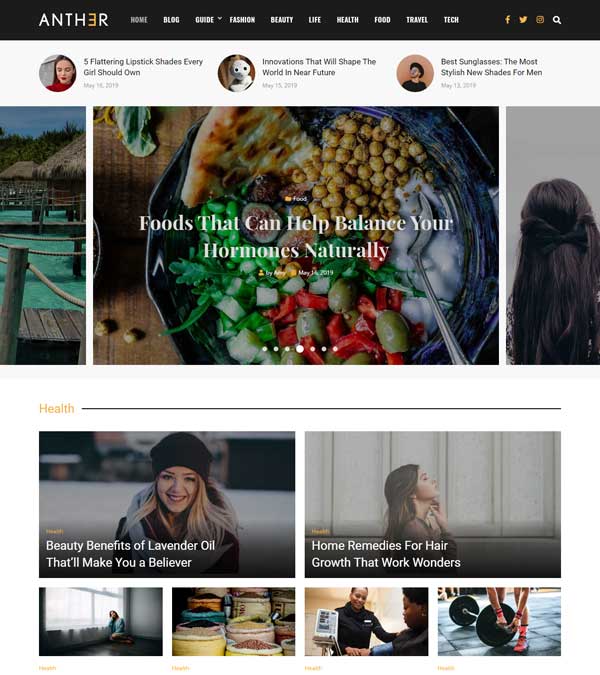The webpage features a navigation bar labeled "Anther," and includes links to sections such as Home, Blog, Guide, Fashion, Beauty, Health, Food, Travel, and Tech. Social media icons for Facebook, Twitter, and Instagram are also present, along with a magnifying glass icon for search functionality.

The main focal point of the page includes a large image of a woman looking down, showcasing her vibrant red lipstick. The accompanying text reads, "Bright Flattering Lipstick Shades Every Girl Should Own." 

Other highlighted sections include various articles and features:
1. "Innovations Always Shape the World: A New Future."
2. "Best Sunglasses for 2023."
3. "The Most Stylish T-Shirts for Men."

The left side of the page displays an image of some canopies or a bridge, set against a backdrop featuring a glass umbrella. 

In the center of the page, there is an article titled "Foods That Can Help Balance Your Hormones Naturally." The image accompanying this article shows a rustic table adorned with an assortment of foods such as pita bread, chickpeas, yogurt, peppers, and greens. 

Additional highlighted tags and categories include Health, Benefits of Lavender Oil, and various home remedies that are claimed to work wonders. 

At the bottom are four square icons, likely quick links or featured categories, although their text is not clearly visible.